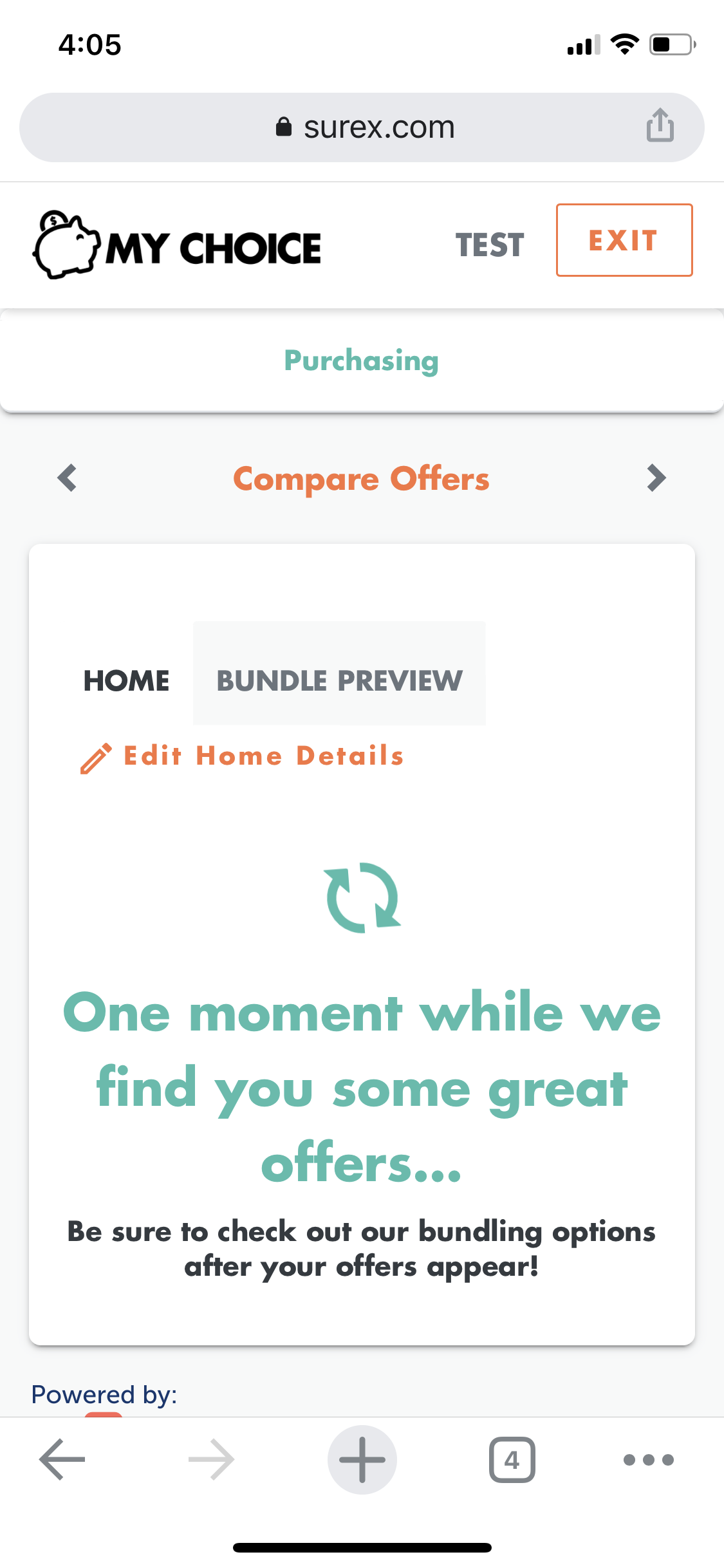This image features a screenshot of a mobile webpage, specifically from the website surex.com, displayed on a cell phone. At the very top, the standard status bar of a phone is visible, including a clock on the left, and the network signal, Wi-Fi signal, and battery meter on the right. Just below this status bar, the web address "surex.com" is prominently displayed.

Immediately beneath the web address, there is a heading labeled "My Choice," accompanied by an icon resembling a piggy bank. Adjacent to this heading are two buttons labeled "Test" and "Exit". Following this section, the text "Purchasing" is written in green, indicating the likely purpose of the page.

Below the "Purchasing" text, in orange, is a section labeled "Compare Offers," flanked by navigation arrows indicating previous and next options. Further down, we see additional navigation options labeled, "Home," "Bundle Preview," and "Edit Home Details".

The central part of the image suggests that the page might be in a loading state. It reads in green, "One Moment While We Find You Some Great Offers." Beneath this, in black text, there's a prompt encouraging users: "Be Sure To Check Out Our Bundling Options After Your Offers Appear."